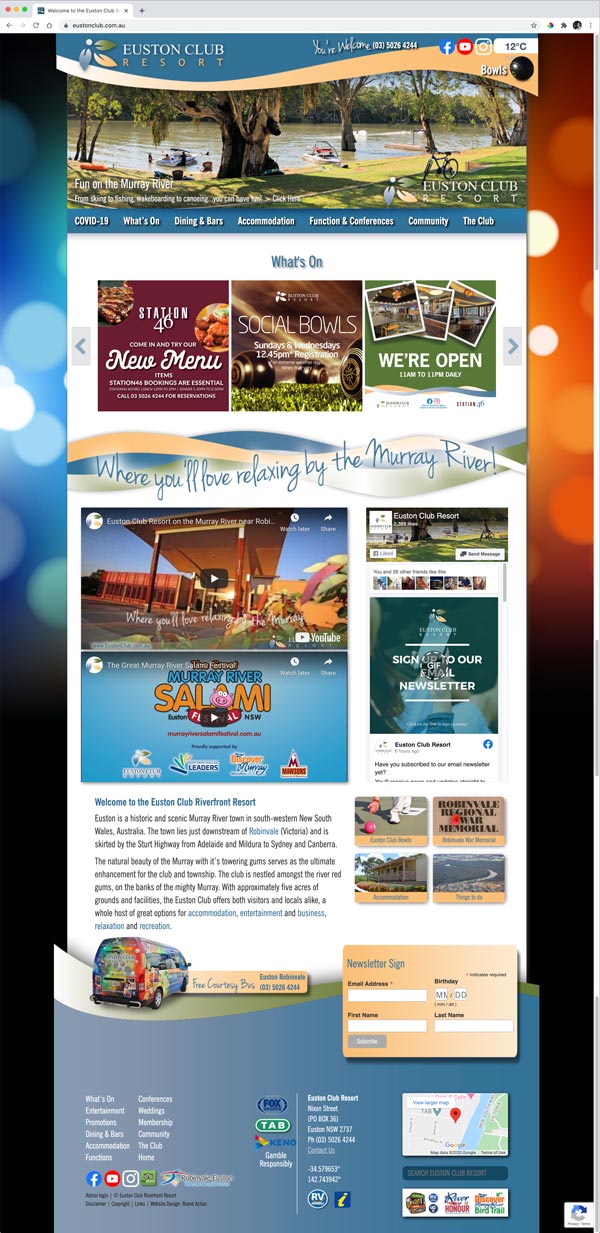At the very top, there is a grey bar displaying red, yellow, and green icons. Below it, the text "Welcome to the Houston Club" is prominently featured, accompanied by a logo with blue, yellow, and green leaves. The website "houstonclub.com.au" is visible along with the text "Houston Club Resort."

Contact details such as "03050264244" and social media icons for Facebook, YouTube, and Instagram are also displayed. Bowls are shown in the image, and at the center, there is a picturesque lake surrounded by grass, trees, and boats.

The caption indicates various activities like skiing and fishing available on the Murray River. It also mentions sections for COVID-19 updates, dining and bars, accommodation, functions and conferences, community activities, and club events.

One of the announcements reads, "Station 46: Come and try our new menu items. Station bookings are essential. Open Sundays and Wednesdays at 12:45 PM. Operating hours are 11 AM to 11 PM daily." The text highlights "Murray Love Relaxing by the Murray River" and encourages visitors to "sign up to our email newsletter." 

Another advertisement features "Murray River Salami" and invites people to "Welcome to the Houston Club Riverfront Resort," located in Houston's historic city, a Murray River town in southwestern New South Wales, Australia. The town lies just south of the Victoria River and is easily accessible from the Adelaide-Meadow to Sydney-Cambria highway.

Described as a natural beauty spot, the Murray River's towering glaciations make it a popular destination for both the club and the township. Nestled on the banks of the mighty Murray, the Houston Club spans approximately 5 acres, offering optimal accommodation, entertainment, business opportunities, relaxation, and recreational activities to both visitors and locals.

The newsletter signup section invites users to provide their email address, first name, birthday, and last name. The final list summarizes current events, entertainment, and promotions happening at the Houston Club.